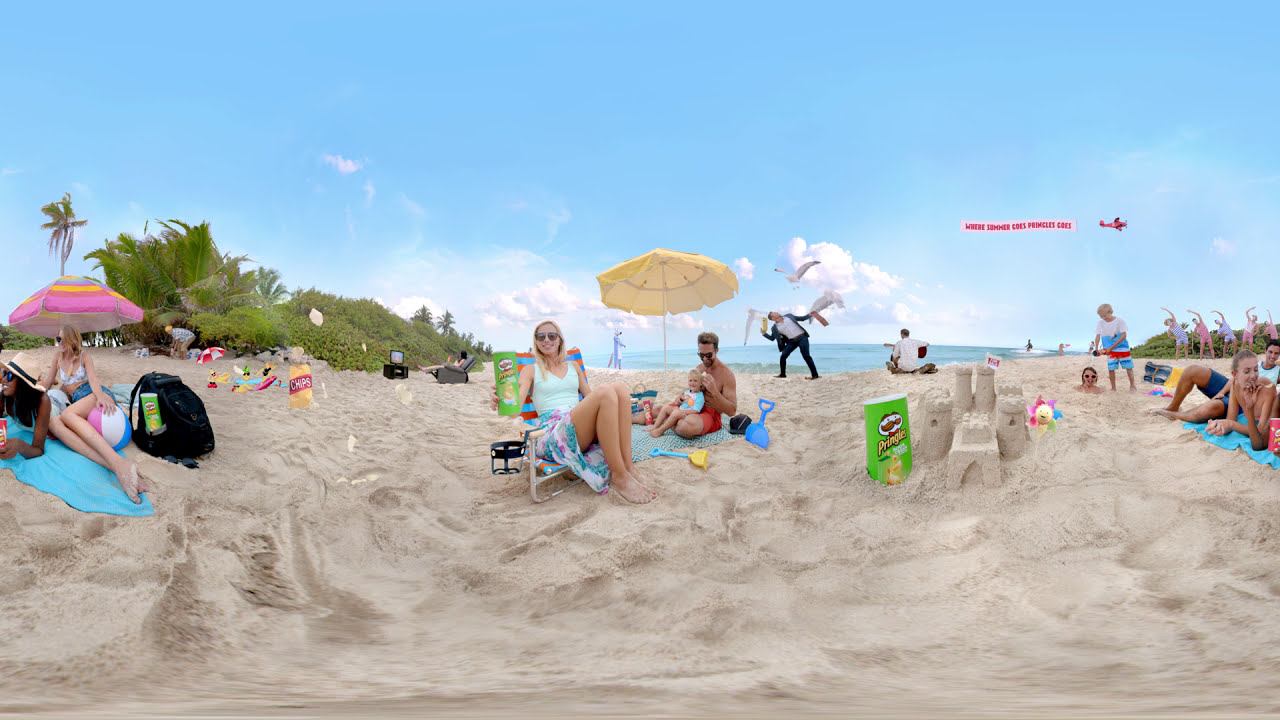This is a curved, slightly distorted panoramic photograph of a busy beach scene, created using a fisheye filter that gives it a 360-degree view. The light gray sand is populated with both men and women who are engaging in various activities such as sitting, standing, or relaxing on towels. The beach is littered with several packets of chips, particularly Pringles, which play a prominent role in the image. In the center, a fair-skinned blonde woman wearing sunglasses, a light blue shirt, and a flowery dress, holds up a green can of Pringles towards the camera—a clear nod to the advertisement theme. 

Above her, a plane flies with a banner reading, "Where summer goes, Pringles go." In the background, people are enjoying their time on the beach, celebrating, and even animated Pringles chips join in the fun. On the left side of the image, a small tropical oasis stands out amidst the sandy beach, adding a quirky element. Nearby, two people under a pink umbrella have a black backpack with a Pringles can beside them. 

Further to the right, you can find a Pringles can partially buried in the sand next to a sandcastle. The blue sea stretches out in the front, contrasting with the light blue sky dotted with white clouds. In the backdrop, green trees and plants provide a lush boundary to the beach scene, highlighting the advertised message of summer fun with Pringles.